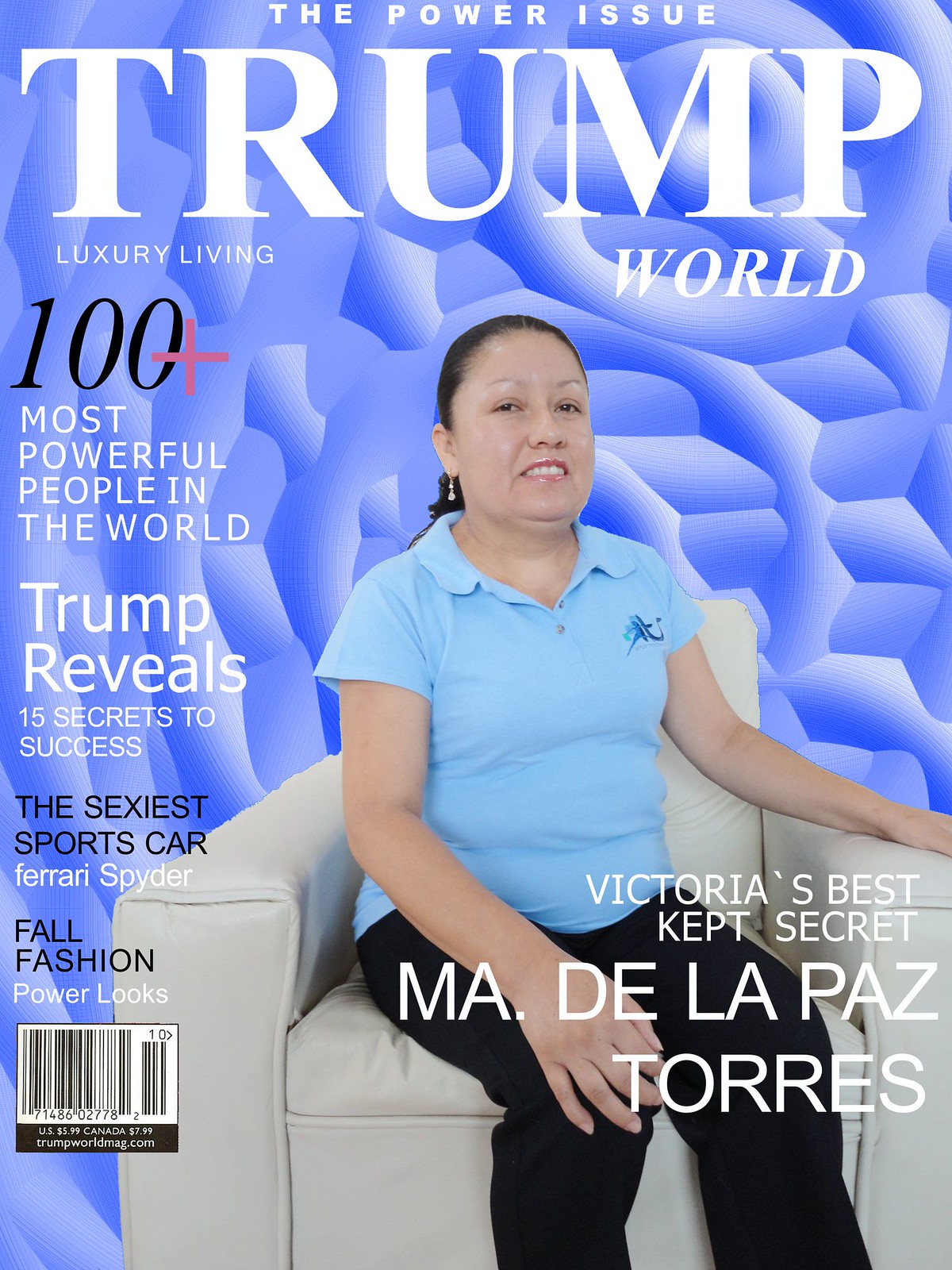The magazine cover features a striking blue, abstract background composed of puffy geometric symbols. Seated on a large, leather chair that resembles a comfortable recliner, a Caucasian woman with her black hair pulled back into a ponytail is present. She is dressed in a blue polo shirt with a logo on the left side, paired with black pants. Her dark eyes look confidently at the camera.

At the very top of the cover, in small white capital letters, the text reads "THE POWER ISSUE." Below this, "TRUMP" is prominently displayed in large white capital letters, followed by the word "WORLD" in slightly smaller print. To the left of the woman, the text "LUXURY LIVING" is written alongside various feature highlights, including "100+ Most Powerful People in the World," "Trump Reveals 15 Secrets to Success," "The Sexiest Sports Car: Ferrari Spider," "Fall Fashion: Power Looks," and "Victoria's Best Kept Secret: M.A. Kiernan De La Paz Torres." Additionally, a barcode is situated towards the bottom left corner of the cover.